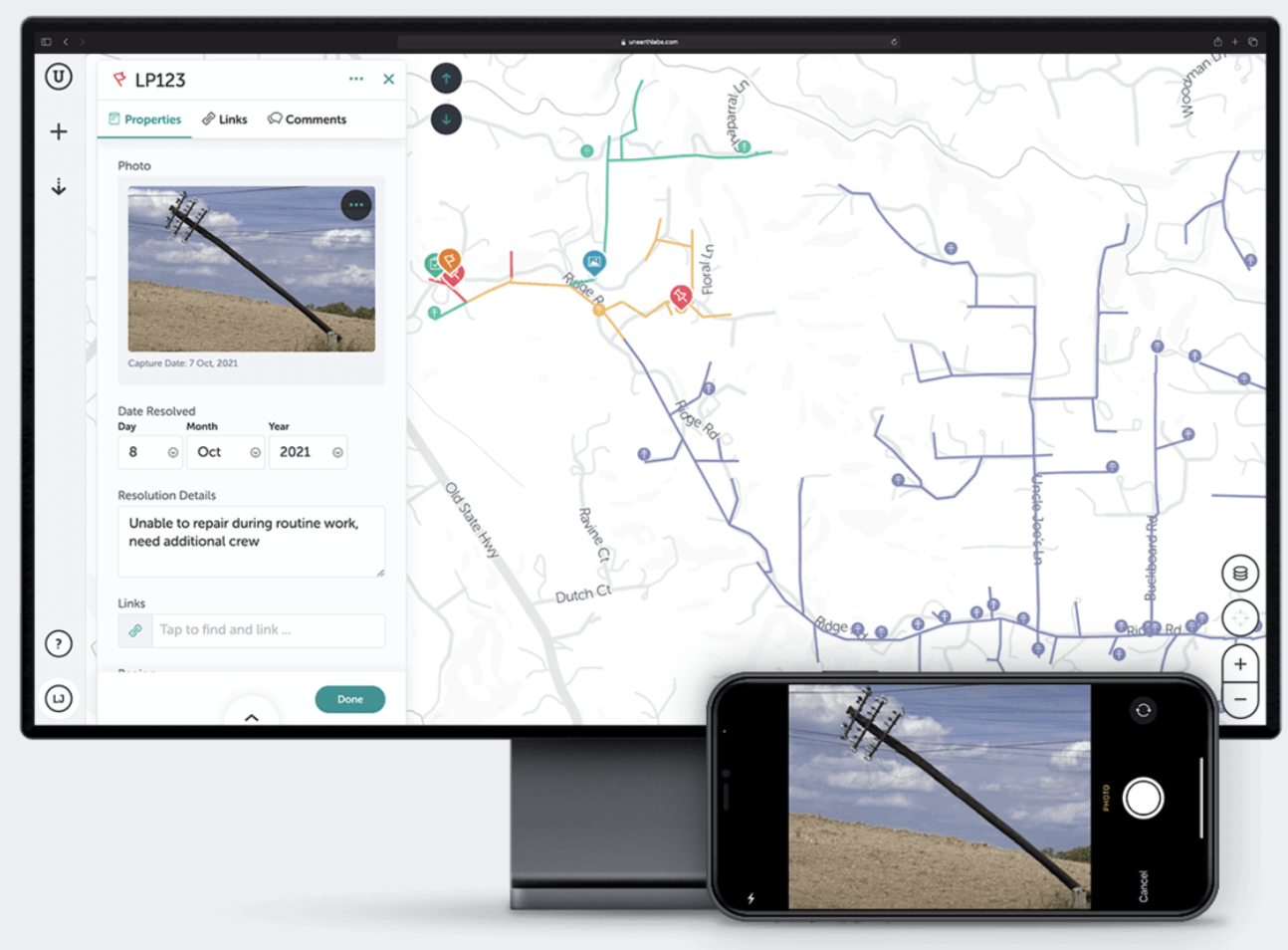The image appears to be a well-crafted advertisement depicting a high-resolution photograph of a computer monitor. The monitor displays a mapping application, possibly intended for utility maintenance or geographic information systems. Unlike typical images taken of computer screens, this photograph is clear and free of rainbow-like pixelation, emphasizing its quality and professionalism.

On the screen, the mapping software shows a detailed map of a city, with various labeled sections including LP123, alongside features such as "Properties," "Links," and "Comments." Within the interface, there is a thumbnail labeled "Photo," showcasing a sandy area with a severely leaning power pole at approximately a 45-degree angle. An annotation on the screen notes, "Date Resolved: October 8, 2021," followed by a status update indicating, "Unable to repair during routine work. Needs additional repairs."

The map view is revisited lower in the image. Adjacent to the monitor on the desk is a sideways iPhone, displaying a larger version of the photo featuring the damaged power pole, reinforcing the area's need for infrastructural attention. The overall setup suggests that this scene is documenting a utility maintenance issue, possibly after a severe weather event such as a tornado. The precise documentation and clear visuals underline the importance of identifying and mapping damages for prompt and effective repairs.